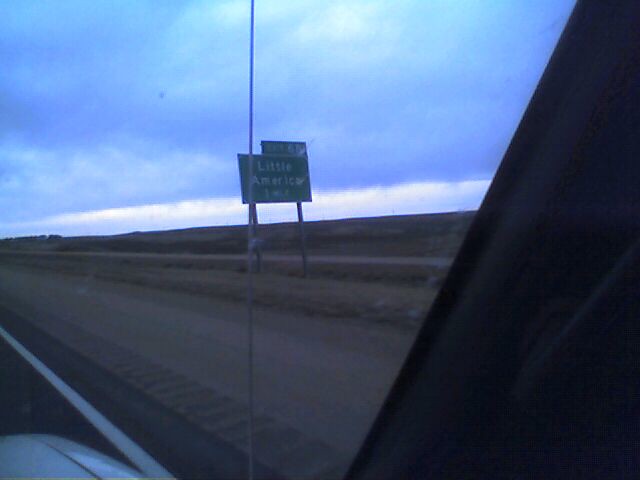In this scenic image, a bright stretch of blue sky is dotted with white clouds, creating a serene backdrop. Prominently featured is a green road sign bearing the words "Little America," supported by two sturdy metal legs anchored into the ground. The scene includes a brown dirt road marked with a single tire track, indicating the path of a recent vehicle. To the left, a tent is partially visible, lending an element of outdoor adventure to the setting. Inside the vehicle, the dashboard appears with a sleek plastic trim on the right side, and the windshield shows only slight traces of dirt with a few specks visible. The horizon is filled predominantly with clouds, enhancing the sense of open space and tranquility.